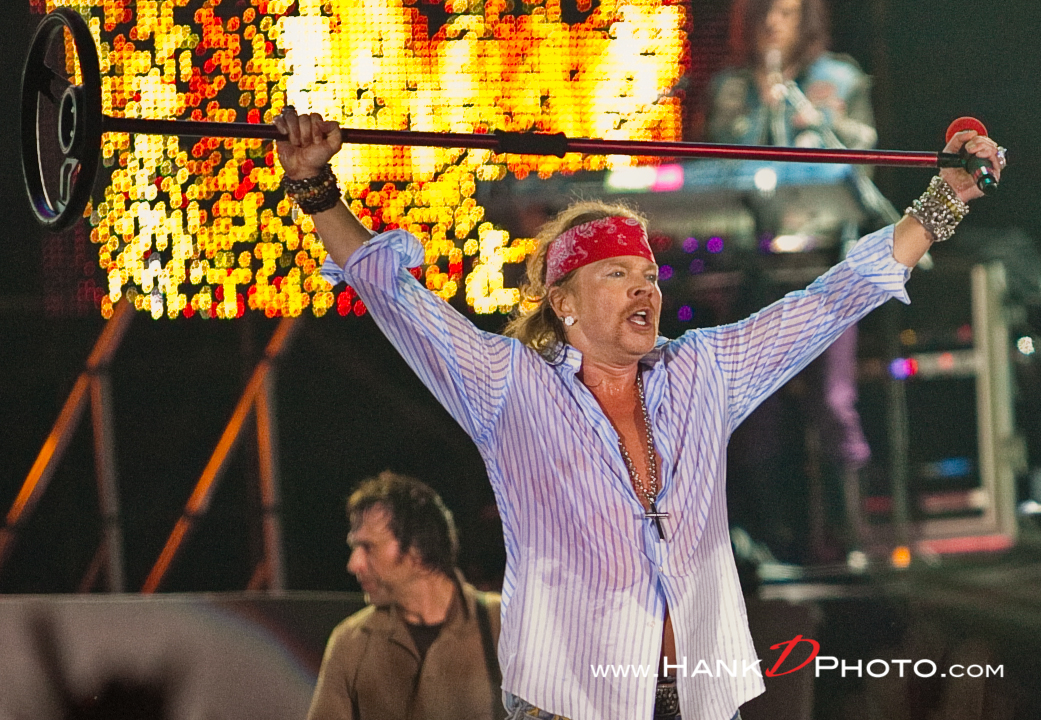In this detailed photograph, Axl Rose, the iconic lead vocalist of Guns N' Roses, is captured energetically performing on stage. Dressed in a white shirt with blue stripes and the top buttons unbuttoned, Axl exudes his signature rockstar charisma. The photo shows him holding a microphone in his left hand and raising the stand above his head with his right hand, appearing as if he's just finished an impassioned yell, his mouth wide open. A red bandana is tied around his head, revealing his long blonde hair. A plethora of bracelets adorns his wrists, and rings gleam on his fingers, adding to his typical flamboyant style. A silver chain with a prominent cross pendant hangs down to his chest. His blue eyes and goatee are highlighted by some makeup, giving him a striking stage presence. In the background, the rest of the band is visible, with one member playing the keyboard and another handling the guitar, surrounded by bright stage lights. The bottom right corner of the image bears the watermark www.hankdphoto.com, adding a professional touch to the photograph.